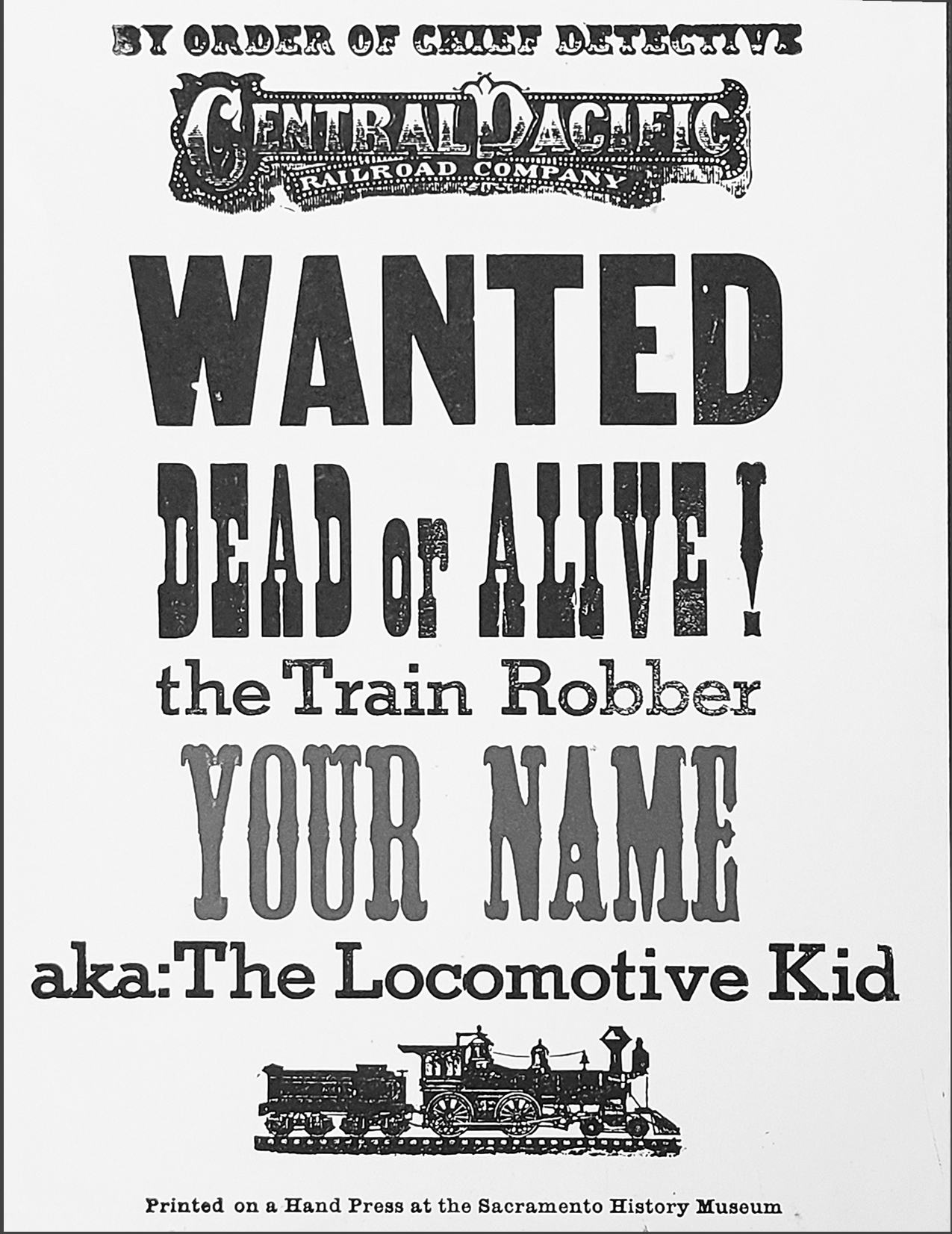This image features an old-fashioned Western-style wanted poster template designed as a birthday party gimmick. The poster, predominantly in black, white, and gray, reads: "By order of Chief Detective, Central Pacific Railroad Company, Wanted Dead or Alive, The Train Robber, [Your Name], aka The Locomotive Kid." Each line is printed in a different font reminiscent of the Wild West, giving it an authentic historical feel. The poster is bordered in black, enhancing its vintage appearance. At the bottom, there is an icon of a train on a track, and in fine print, it states: "Printed on a hand press at the Sacramento History Museum." The text varies in size and style, adding to the aesthetic appeal of this customizable keepsake.